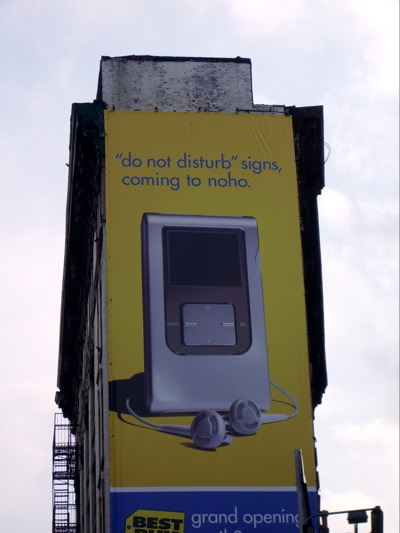The image depicts a large rectangular billboard hanging on the side of a tall brick building, which features a fire escape on the left and a slight flare-out on the right side halfway up. The billboard dominates almost the entire side of the building, against a cloudy sky backdrop. The sign has a yellow background with blue text that reads, "Do Not Disturb, Signs Coming to NoHo." Below the text, there is an old-style, silver and grey mp3 player with a small display screen and buttons, connected to wired earbuds. At the bottom of the billboard, there is a blue horizontal section displaying the Best Buy logo with the words "Grand Opening." A streetlight is also barely visible in the bottom right corner of the image.